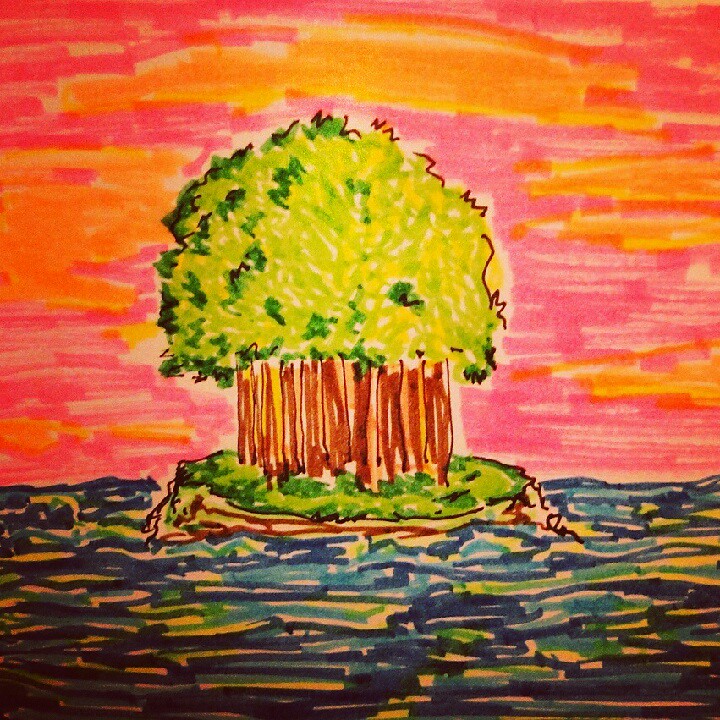This square, marker-style illustration depicts a small, serene island adorned with lush grass and an intriguing tree formation. The trees are drawn in such a way that their trunks appear to merge into a single, large trunk, giving the impression of a unified arboreal structure. The dense foliage at the top is rendered in vibrant shades of yellow and green. The sky above the island is a mesmerizing blend of orange and pink hues, showcasing dynamic brush strokes that add texture and depth. The surrounding water features a captivating gradient of green, light blue, and dark blue, creating a harmonious yet lively contrast with the island.